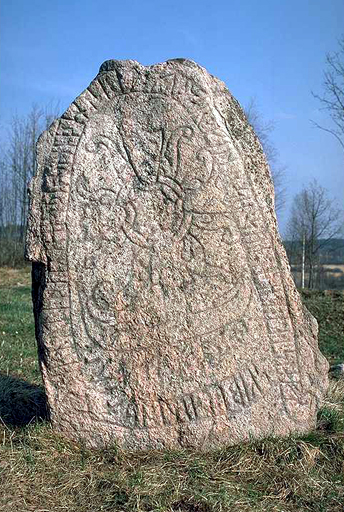This image features an ancient stone monument standing prominently in the center of a grassy field. The stone, weathered by time and elements, shows signs of erosion and chipping, adding to its aged and rugged appearance. Intricate decorative patterns adorn its surface, with what appears to be a sun or star motif in the middle, surrounded by ancient, unreadable text that resembles hieroglyphics. The top of the stone particularly shows signs of wear, suggesting it has endured centuries, possibly even millennia. The monument casts a significant shadow on the bright, sunlit day, adding contrast to the scene. In the background, leafless trees suggest a fall or winter setting, while the bright blue sky enhances the visibility of the stone’s details. The grass field stretches out behind the monument, with hints of farmland further in the distance. The overall atmosphere conveys a sense of ancient history and mystery.